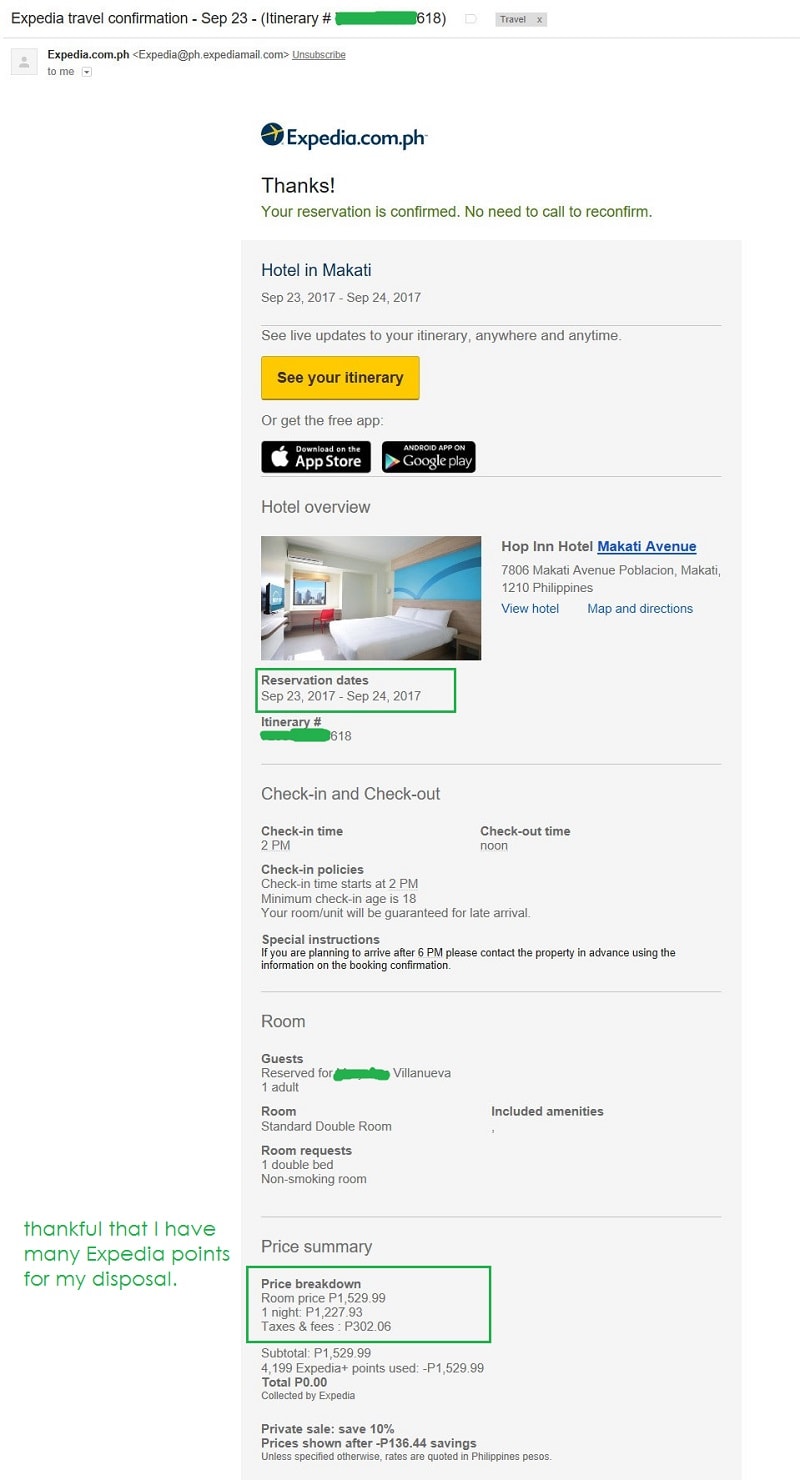**Expedia Travel Confirmation - Detailed Summary**

**Page Overview:**
This confirmation page from Expedia.com.ph features a reservation summary on a clean, white background.

**Headers and Key Details:**
- **Date:** September 23, 2017
- **Itinerary Number:** Ends with 618 (initial digits are obscured by a green line)
- **Reservation Status:** Confirmed with the message "Thanks, your reservation is confirmed. No need to call to confirm."
- **Travel Dates:** September 23, 2017, to September 24, 2017
- **Destination:** Hotel in Makati
- **Live Updates:** Available anytime and anywhere

**Call-to-Actions:**
- **Yellow Box:** "See your itinerary"
- **Promotional Messages:**
  - "Or get the free app" with icons for the Apple Store and Google Play Store

**Hotel Overview:**
- **Room Image:** Displays a mostly white room with minimalistic decor.
  - **Bed Area:** Features pale wood (beech or birch) paneling behind the bed, with a light blue section crossed by a dark blue curved line.
  - **Window View:** Cityscape visible outside the window
  - **Furniture and Fixtures:** Air conditioner above the window, built-in desk by the window, small TV on a bench to the left.

**Reservation Details:**
- **Dates:** September 23rd - September 24th, 2017
- **Check-in Time:** 2 p.m.
- **Check-out Time:** Noon
- **Guest:** One adult, last name Villanueva
- **Room Type:** Standard double room, one double bed, non-smoking

**Expense Breakdown (Green Box):**
- **Room Price:** ₱1,529.99
  - **One night rate:** ₱1,227.93
  - **Deposits and Fees:** ₱302.06
- **Subtotal:** ₱1,529.99
- **Points Used:** 4,199 Expedia Plus points, resulting in -₱1,529.99, covering the total expense
- **Final Total:** ₱0.00
- **Private Sale Discount:** 10% savings after -₱136.44
- **Currency:** All rates are quoted in Philippine Pesos unless specified otherwise

**Additional Note:**
- **Expedia Loyalty:** Comment expressing gratitude for having many Expedia points available

This comprehensive breakdown covers all key details and features visible on the Expedia travel confirmation page. Each piece of information provides an understanding of what the user sees at a glance.